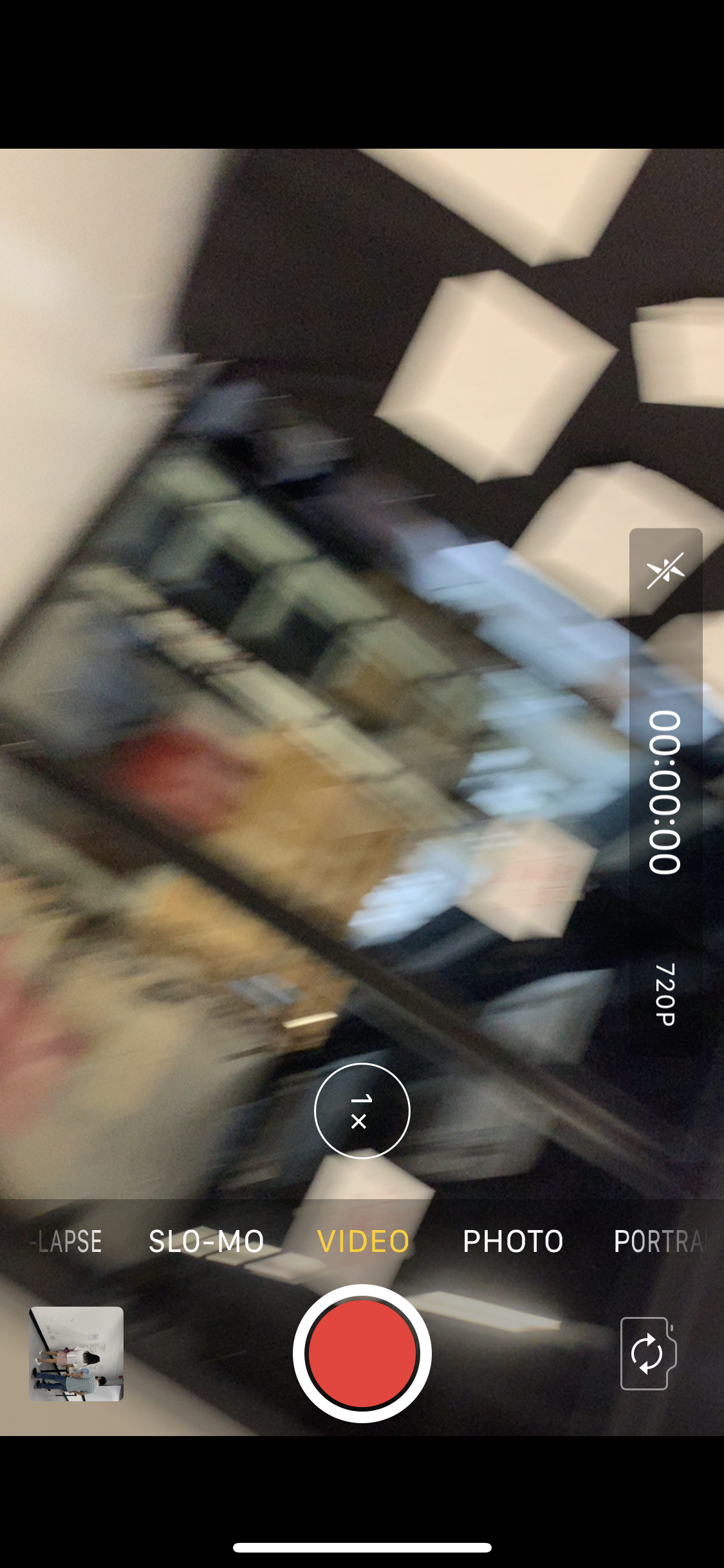The image is a screenshot from a mobile phone's camera application, poised either to take or in the process of recording a video, as indicated by the red recording button at the bottom. The 'Video' mode is selected among options like 'Lapse,' 'Slo-mo,' 'Photo,' and 'Portrait.' In this interface, the '1x' zoom option is active, and symbols such as the flash icon, a '000' counter, and '720p' resolution appear on the right side of the screen. 

The main background is very blurry, obscuring clear details but suggesting the interior of a convenience store, possibly near the entrance or cooler section, given the presence of reflective glass and vague outlines of stacked merchandise. Bright, indistinct colors—white, blue, green, red, and yellow—are scattered through the view. 

In the bottom left corner, there’s a small tilted thumbnail of a previous photograph showing a man and a child standing in what seems to be a white hallway, facing a wall. On the very bottom right, there's an icon of a camera with two arrows around it, indicating a switch camera function. Overall, the screenshot captures a moment of setting up for a video with a partially visible, nondescript environment.